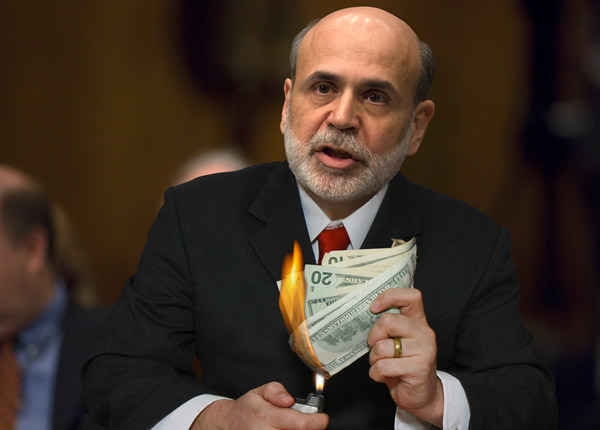In this striking image, a bald politician or spokesperson is captured mid-speech in what appears to be a provocative demonstration. He has a distinctive look with a white beard encircling the sides of his head and connecting to his facial hair. Dressed in a dark suit complemented by a white undershirt and a red tie, he holds a stack of 20-dollar bills along with other denominations in his left hand. In his right hand, he grips a lighter, actively igniting the money as part of his protest or demonstration. His mouth is open as he speaks, adopting a neutral expression that conveys neither anger nor happiness. The blurred figures in the background glance to the right, seemingly focused on something off-screen, while the wooden backdrop suggests the setting is inside a rustic building or chamber. This powerful image encapsulates a moment of defiance or statement about political or economic issues.